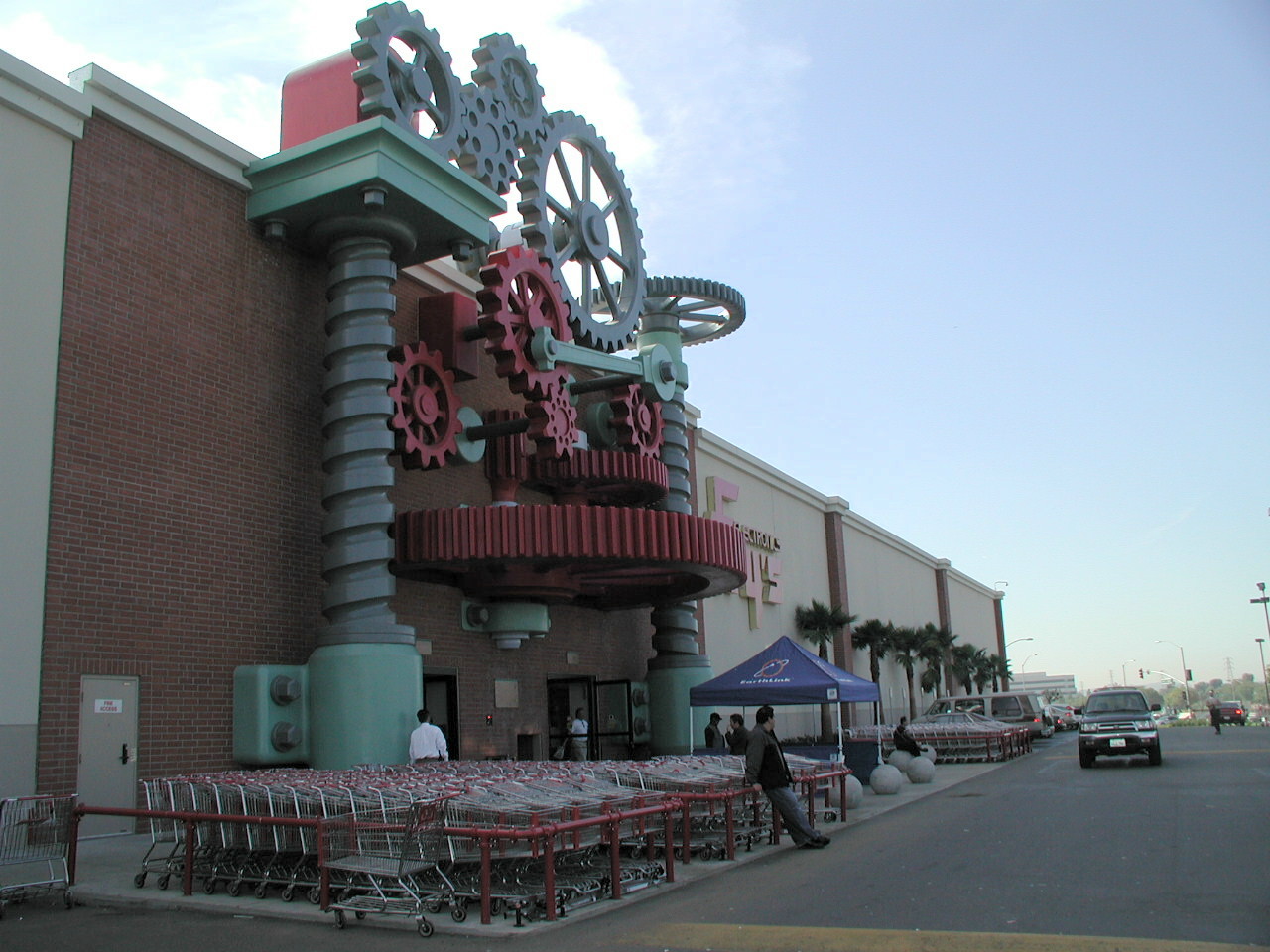This photograph, taken during the daytime with crystal-clear imaging, captures a vivid and detailed urban landscape. Dominating the upper portion of the image is a light blue sky, accentuated by fluffy white clouds. Below, a glimpse of a black concrete roadway can be seen, along with several darker-colored vehicles. The scene features trees juxtaposed against a building, which is divided into a brick section and a tan section.

In front of the building, a cart corral area made of red metal houses numerous silver and red shopping carts. The most striking element of the photograph is the enormous clockwork-like structure affixed to the brick portion of the building. This intricate display features variously colored cogs: silver ones at the top, red ones interspersed throughout, and a prominent giant red cog at the bottom that appears halved. This cog is bordered by green structures and flanked by two enormous green columns with gray centers. The brick portion of the building also includes black doors, adding to the rich details in this vibrant urban snapshot.